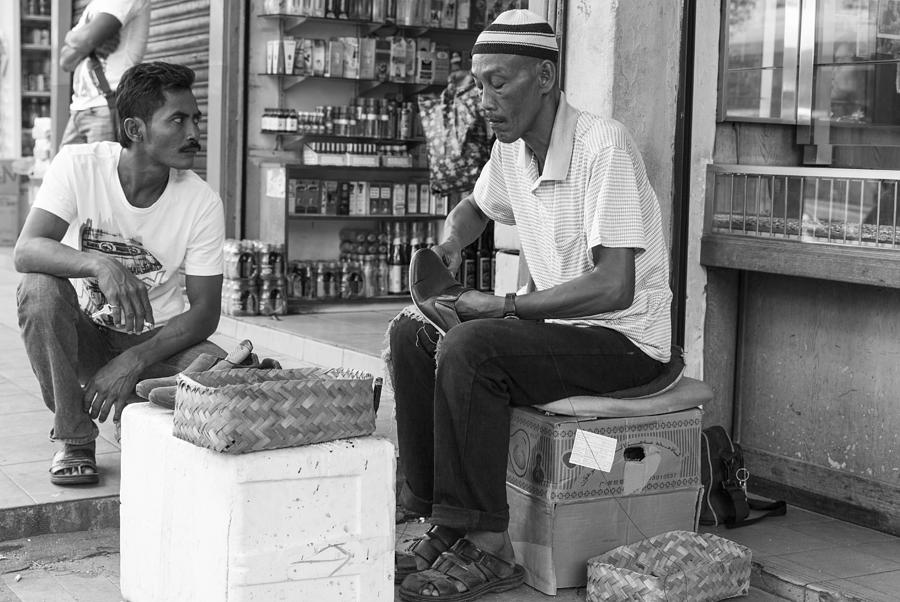This black-and-white photograph captures a bustling street scene, seemingly in a South Asian locale, depicting two men positioned prominently in front of an open storefront. The man at the center, who has a darker complexion, sits on a decorated stool with a cushion. He wears a knit hat with black and white stripes, a striped polo shirt, dark pants, and sandals. His focus is on a shoe he is repairing or polishing, using tools from a white box in front of him. This box also supports a wicker basket and another pair of shoes. To his left, another darker-skinned man with short hair and a mustache crouches down, observing the shoemaker intently. He’s dressed in a white t-shirt with a design, denim jeans, and sandals. The backdrop reveals an open shop door with shelves stocked with bottles and other merchandise, suggesting a lively marketplace setting. In the background, a third person with crossed arms stands partially visible, adding to the scene's dynamic atmosphere.